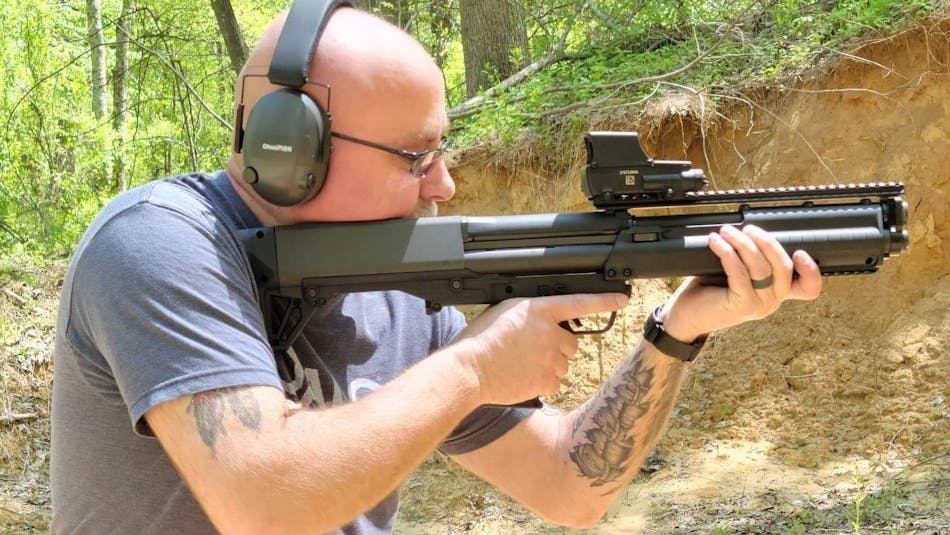The image features a bald man in a light gray t-shirt, intricately decorated with tattoos on his upper right arm and left lower arm. He stands in the foreground of a forested area, near a dirt cliff. The man has on glasses and is wearing black ear protection headphones, indicating he might be at an outdoor gun range. He is holding a large, semi-automatic rifle up to his shoulder, aiming through the scope, eyes focused intently. He sports a black watch and a black wedding ring on his left hand, suggesting his dedication to both time and marital commitment. The scene behind him is vibrant with green trees and leafy foliage, with a tan, sandy dirt area enhancing the mountainous, wooded backdrop. No other individuals are visible, and the overall atmosphere is one of solitary concentration amidst nature.